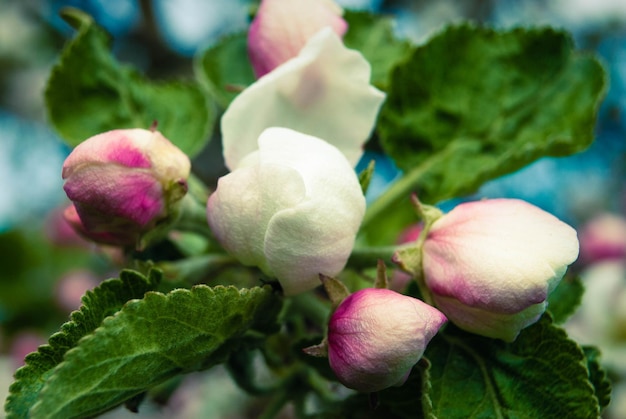This close-up photograph captures the intricate beauty of a flowering plant, likely nestled among various bushes. The image focuses on five or six broad, spinach-green leaves radiating in different directions, framing a cluster of five budding flowers. At the center, two nearly white, rose-like buds with just a hint of pink begin to unfold, while the three surrounding buds display more prominent pink hues near their bases. The delicate buds, resembling small tea roses or possibly tulips, exhibit a pearlescent quality that suggests they are on the verge of blooming. The background is a soft blur of green and blue, hinting at foliage and possibly the sky, contributing to the well-lit, sunny ambiance of the scene.